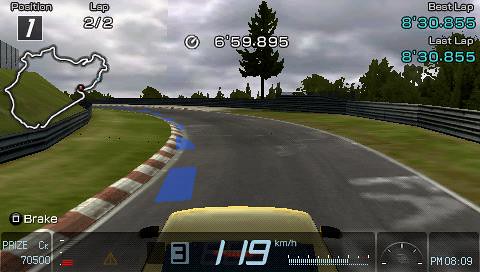The image appears to be a screenshot from an auto racing video game. At the bottom of the screen, the speed is displayed as 119 kilometers per hour. Other dashboard elements indicate the time in PM and a variety of other data, likely simulating a heads-up display on the windshield or the speedometer area of the vehicle. The road ahead curves gently, marked by alternating red and white striped lines on the left side and a grassy verge. Beyond the road, an expanse of trees dot the horizon. On the right side, a green grassy area transitions into a silver barrier wall, presumably for safety to prevent the car from veering off the track. The sky above is overcast, mostly covered in gray clouds with a few rays of sunlight breaking through.